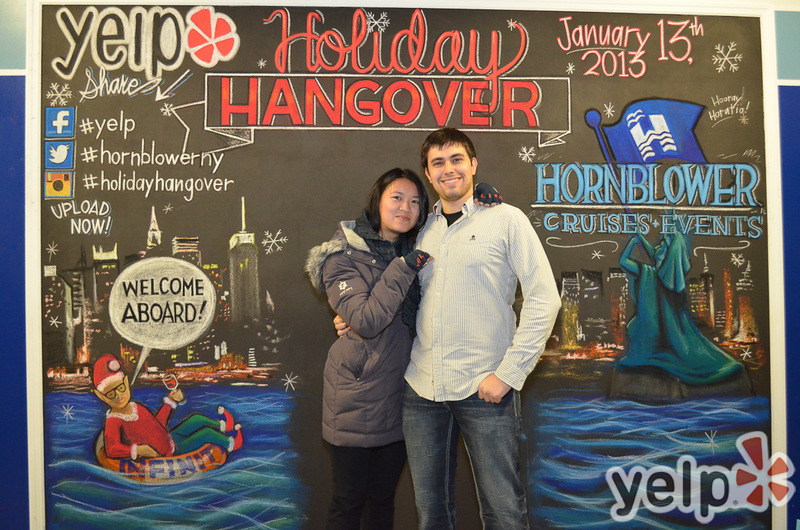A couple is posing for a photograph in front of a vibrant billboard that loudly states "Holiday Hangover" in bright red letters. The man is dressed in a light cream striped shirt and blue jeans, while the woman wears a winter jacket with a fur-rimmed hood and black pants. The backdrop showcases a city skyline with a lake in the foreground. To the left of the billboard, there is a Yelp logo accompanied by social media hashtags for Yelp and "holiday hangover" on platforms like Facebook, Twitter, and Instagram, each marked with their respective logos. An elf, sitting on a life raft that reads "Welcome Aboard," adds a whimsical touch to the scene. On the right side of the billboard, the date "January 13, 2013" is prominently displayed above the Hornblower Cruises and Events logo, which features a statuesque woman holding a blue flag with a white "H" and the text "Hornblower Cruise Events."